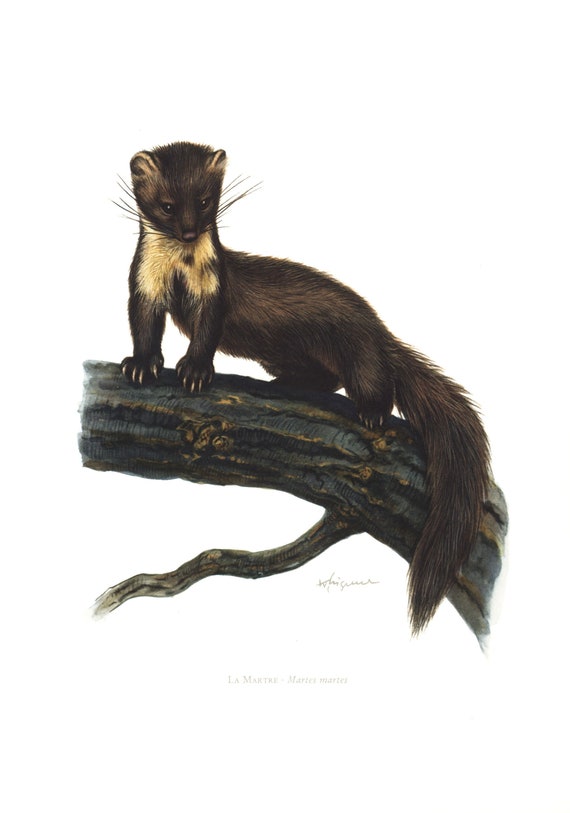This highly detailed illustration depicts a marten, a small woodland animal related to the weasel family, positioned on a nearly black tree branch, which is part of a trunk artistically cut off on both ends to direct attention to the animal. The marten has dark brown fur with a distinctive lighter, blonde or white patch on its chest, resembling a bib. It possesses large, prominent whiskers, small round ears, and long claws on its feet. The marten is facing sideways on the branch, but its front legs and face are turned towards the viewer, with the gaze directed downward. The animal features a long, bushy tail nearly the length of its body and dark, expressive eyes. The illustration lacks a definitive outline, blending seamlessly with the white background. Beneath the image, small, faint writing reads "La Martre, Martes Martes," indicating the species and possibly the artist's signature.